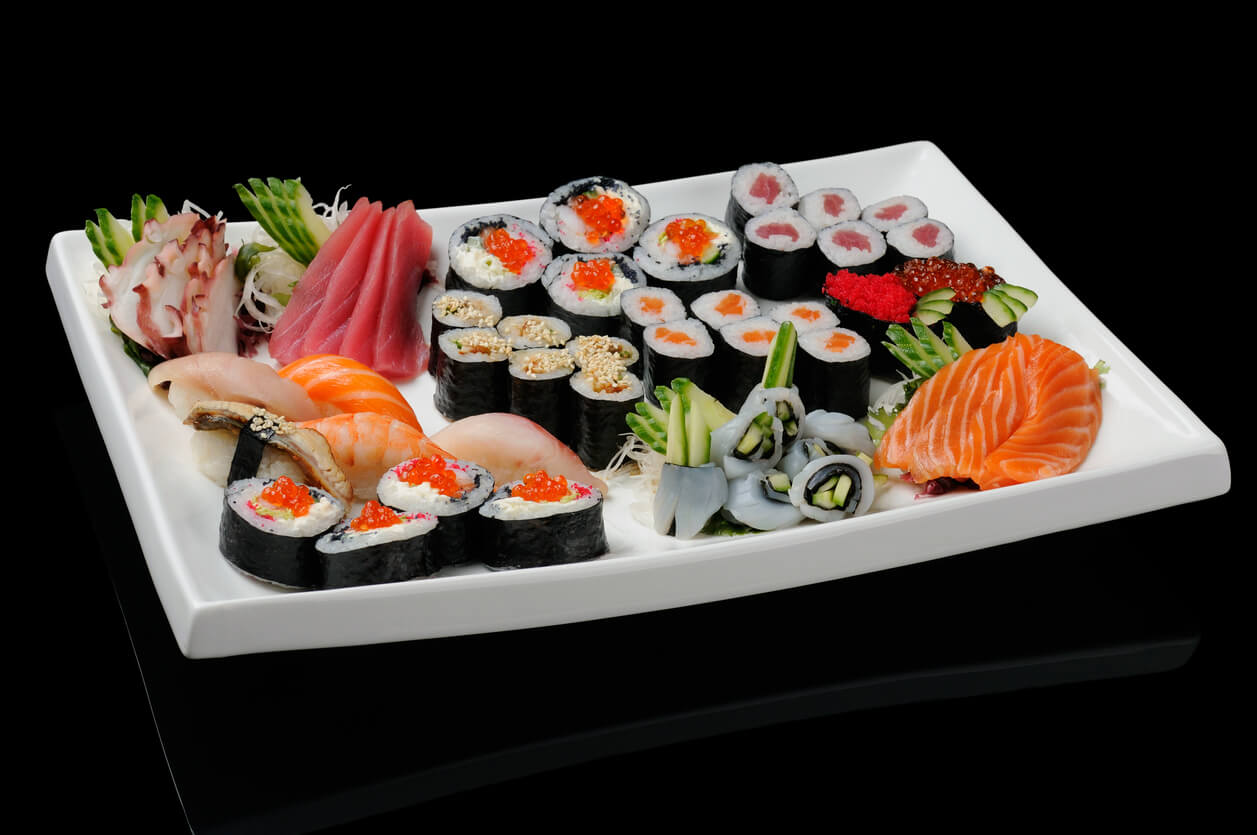The image features a meticulously arranged assortment of sushi on a white, rectangular plate with slightly upturned edges. The plate rests on a highly reflective black surface, creating a striking contrast and mirror-like effect on the bottom. The sushi is artfully divided and organized by type, presenting a vibrant array of colors and textures. 

Starting at the bottom left corner, there are four California rolls adorned with bright orange fish roe. Adjacent to these are four wrapped prawn sashimi pieces. Moving to the top left corner, thin slices of raw octopus rest on a bed of sliced cucumbers, while beside them lie another set of four slices of reddish fish, similarly laid on cucumber and cabbage. In the center, various California rolls are arranged, including six small rolls with sesame seed toppings and another six rolls that may contain carrot. Below these is a piece of unidentifiable, white and translucent seafood wrapped around cucumber slices.

In the bottom right corner of the plate, salmon sashimi slices occupy another cucumber bed. The upper middle section features four larger California rolls topped with bright orange roe and a creamy filling. Capstoning the far right of the plate are two battleship-style sashimi pieces, one topped with red and the other with orange roe, both garnished with sliced cucumber. Finally, the top right corner contains another set of six small California rolls, these with tuna filling. The overall presentation exudes a harmony of seafood varieties, including salmon, shrimp, octopus, and fish roe, complemented by vivid green cucumbers and other vegetables.